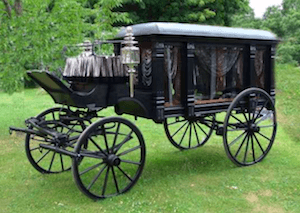This detailed photograph showcases a Victorian-era, black-painted stagecoach, historically used to carry coffins. It is prominently positioned on a well-manicured grassy area with clover patches, under the sunlight. The coach features large wagon-style wheels and is constructed mainly of black iron, presenting an elegant design for its time. Both sides of the coach are adorned with glass viewing panels, draped with intricate brown and white mesh curtains that add to its somber yet sophisticated appearance. Flanking the seat at the front are two clear glass lanterns, framed by silver embellishments. In the background, the lush lime-green trees complement the vibrant grassy setting, providing a serene and picturesque backdrop that contrasts with the coach's dark and solemn presence. The sunlight blurs slightly on top of the carriage, adding a touch of ethereal beauty to the scene.